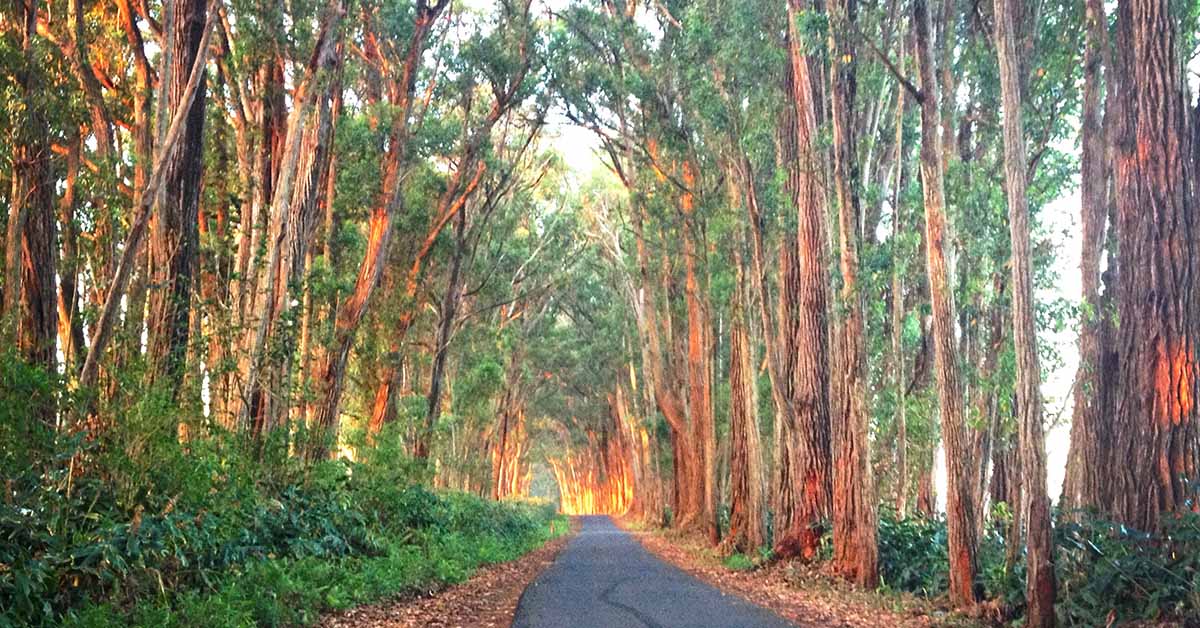This photograph captures a serene, sunlit forest scene with a narrow, smooth concrete road meandering through a dense thicket of tall, green-leafed trees. The road, which could be a bicycling path or a walkway, stretches into the distance, slightly undulating up and down. Lush green grass, bushes, and shrubs flank both sides of the road, adding to the natural beauty of the setting. The ground is sprinkled with a few fallen leaves, hinting at a cool but not wintry time of year. While the location and exact season are unspecified, the daylight and lack of snow suggest a bright, clear day, likely in a temperate climate. The entire landscape exudes tranquility and is devoid of people and animals, focusing solely on the pristine beauty of nature.